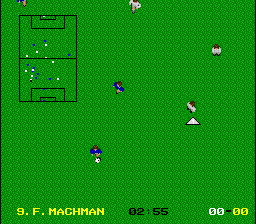The image portrays a scene from a video game featuring a sports match between two teams, one in blue uniforms and the other in white. The background shows a detailed playing field with athletes engaged in what appears to be an ongoing game. The scoreboard at the bottom displays "9F Mach Man," indicating the game's title or the player's identity. The time on the display reads "02:55," possibly marking the duration of the match so far. There are also four zeroes to the immediate right of the timer, which might represent the current score or another in-game metric. On the left side of the scoreboard, small round dots are visible, likely symbolizing the players from each team. In the image's focal point, three athletes in white shirts and two in bright blue shirts are seen moving around the field, suggesting active participation in the sports event within the game.